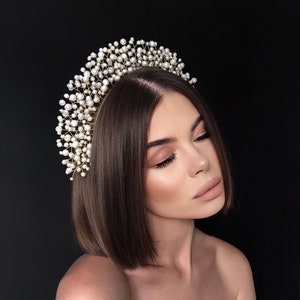This detailed headshot captures a woman with her eyes closed and head gently tilted to the right. She sports silky, straight brown hair that falls gracefully to her shoulders. Her makeup is meticulously done, featuring black faux eyelashes, a neutral shade of lipstick, and subtle shading on her cheeks. Notable is her large tiara-like headband adorned with numerous small white flowers or pearl-like ornaments, giving an impression of a regal crown. Photographed against a dark black or gray background that enhances the contrast, the image focuses on her bare shoulders and neck, devoid of any visible clothing.